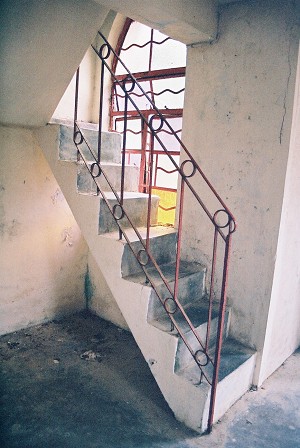This photograph captures the interior of an abandoned, older structure, potentially even a lighthouse. The building, composed of worn-out white stone or concrete, features a steep, multi-level staircase made of identical material. The staircase consists of seven steps and is lined with artistic, circular-patterned red metal railings, which have a somewhat rusty appearance. The floor beneath is covered in dust, dirt, and litter, emphasizing the building’s state of disrepair. 

Dominating the right side of the image is a tall, vertically-oriented window topped with a dome-like arch, and framed with the same red metal as the staircase rails. While it is difficult to determine if panes still reside in the window, the lingering metal bars suggest a functional shutter design, adding an artistic touch to the otherwise decayed environment. The light flooding in through the window highlights the chipped paint on the dirty walls, enhancing the sense of abandonment within this bright yet neglected space.